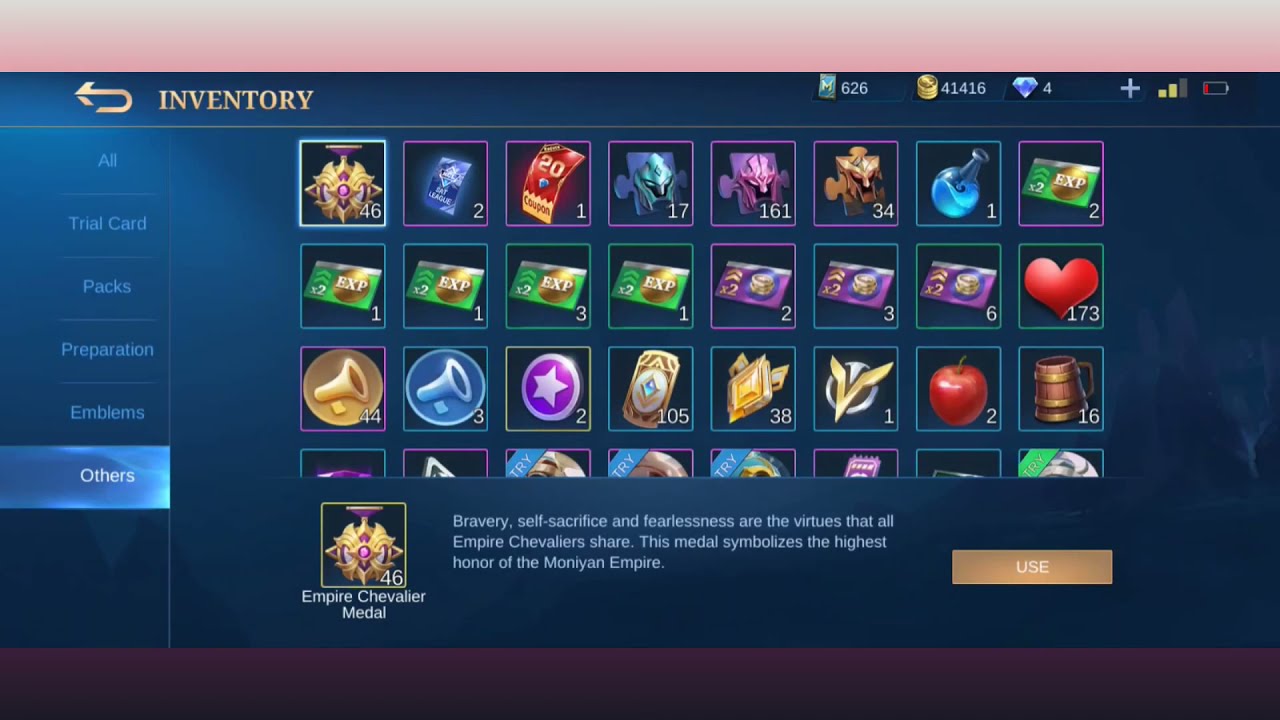The image is a screen grab from a mobile video game, captured while the player is on the inventory page. The main screen has a dark navy blue background, bordered horizontally on the top with a pinkish hue and on the bottom with burgundy. At the very top left, "Inventory" is written in gold text next to a looped back arrow, indicating navigation. On the top right corner, small icons display a very low battery life and Wi-Fi signal status.

Central to the image is a 4x8 grid showcasing various inventory items, each represented by unique icons and accompanied by numerical indicators in the bottom right of each square, signifying the quantity of each item. The inventory shows diverse items such as credit cards, hearts, masks, medals, apples, drinking mugs, potions, and includes specific indicators like gold coins (41416), diamonds (4), and an icon labeled with the number 626.

On the left side of the screen, a vertical text menu allows players to filter inventory items under categories like "All," "Trial Card," "Packets," "Preparation," "Emblems," and the currently highlighted "Others" category, which is marked in a lighter blue.

At the bottom center of the image, descriptive text details a highlighted item: the "Empire Chevalier Medal". It reads: "Bravery, self-sacrifice, and fearlessness are the virtues that all empire chevaliers share. The medal symbolizes the highest honor of the Monian Empire." To the right of this description, there's a brown square button labeled "Use," suggesting the player can select and use this item.